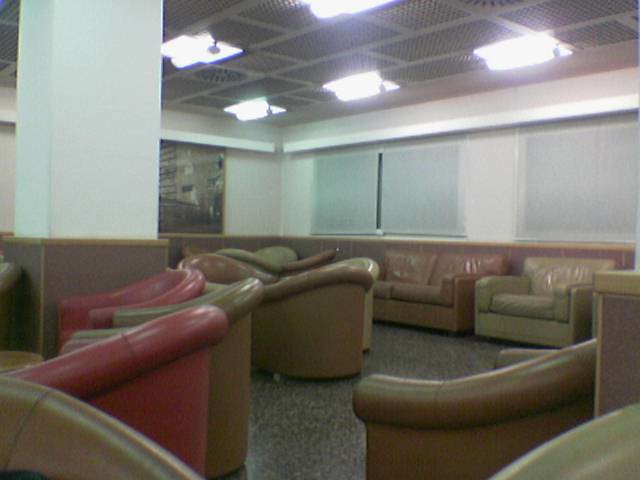The image depicts an indoor setting, likely within a commercial environment, with characteristics that suggest it could be a furniture store or an airport lounge. The room features a patterned hard floor consisting of multiple colors. The walls are cream-colored adorned with pull-down blinds in a light shade. Amidst the plethora of furniture, various seating arrangements include tub chairs and two-seater sofas, all upholstered in a shiny, leather or faux leather material. The furniture is spread out across the room and comes in an assortment of colors including red, brown, beige-green, pea green, light blue, white, and tan. There is a large square pillar emerging from the ground near the left edge of the image and a section of the wall forming a corner off in the distance. The ceiling is equipped with large, shiny fluorescent lights. Additionally, there’s an ambiguous feature to the left which could either be a window or a piece of artwork. No text is visible in the entirety of the photo.